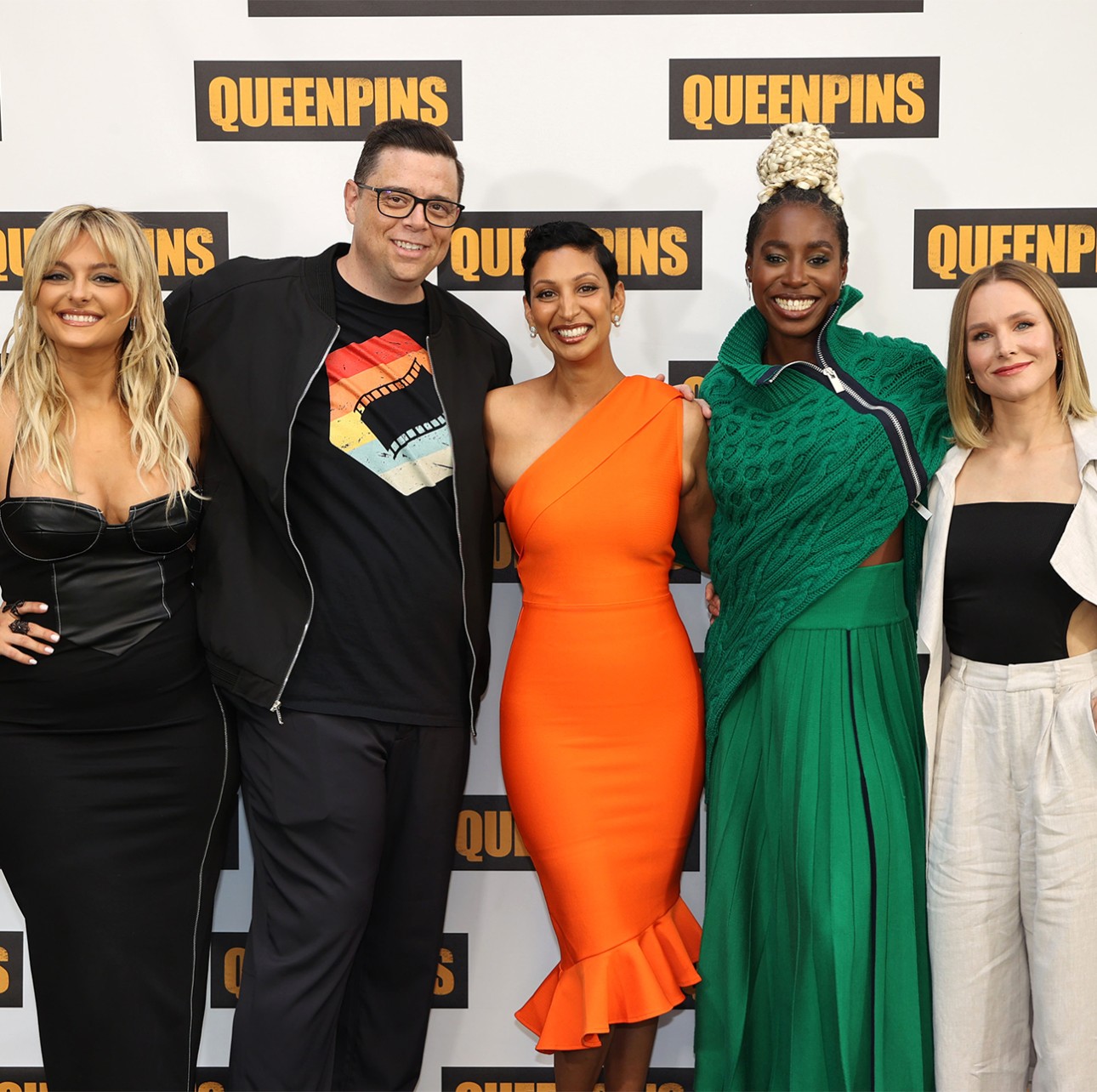In this photograph, a group of five individuals, likely celebrities, are posing in front of a white wall adorned with consistently spaced black signs displaying the words "Queen Pins" in golden yellow ink. From left to right, the lineup begins with a smiling, 30-ish blonde woman in a low-cut, bodycon black dress, her hand confidently resting on her hip. Next to her stands a 40-ish man dressed entirely in black, featuring a black T-shirt adorned with a Pride label in a film strip design and a matching unzipped jacket and pants. To his right is an Indian woman around 40, elegantly dressed in an orange bodycon dress. Beside her, a black woman, positioned slightly sideways, stands out in an all-green ensemble, including a matching jacket. Finally, on the far right, a blonde woman with hair parted in the middle sports a casual, yet stylish white linen pantsuit paired with a black halter top. All five individuals are smiling, exuding a festive and celebratory vibe.